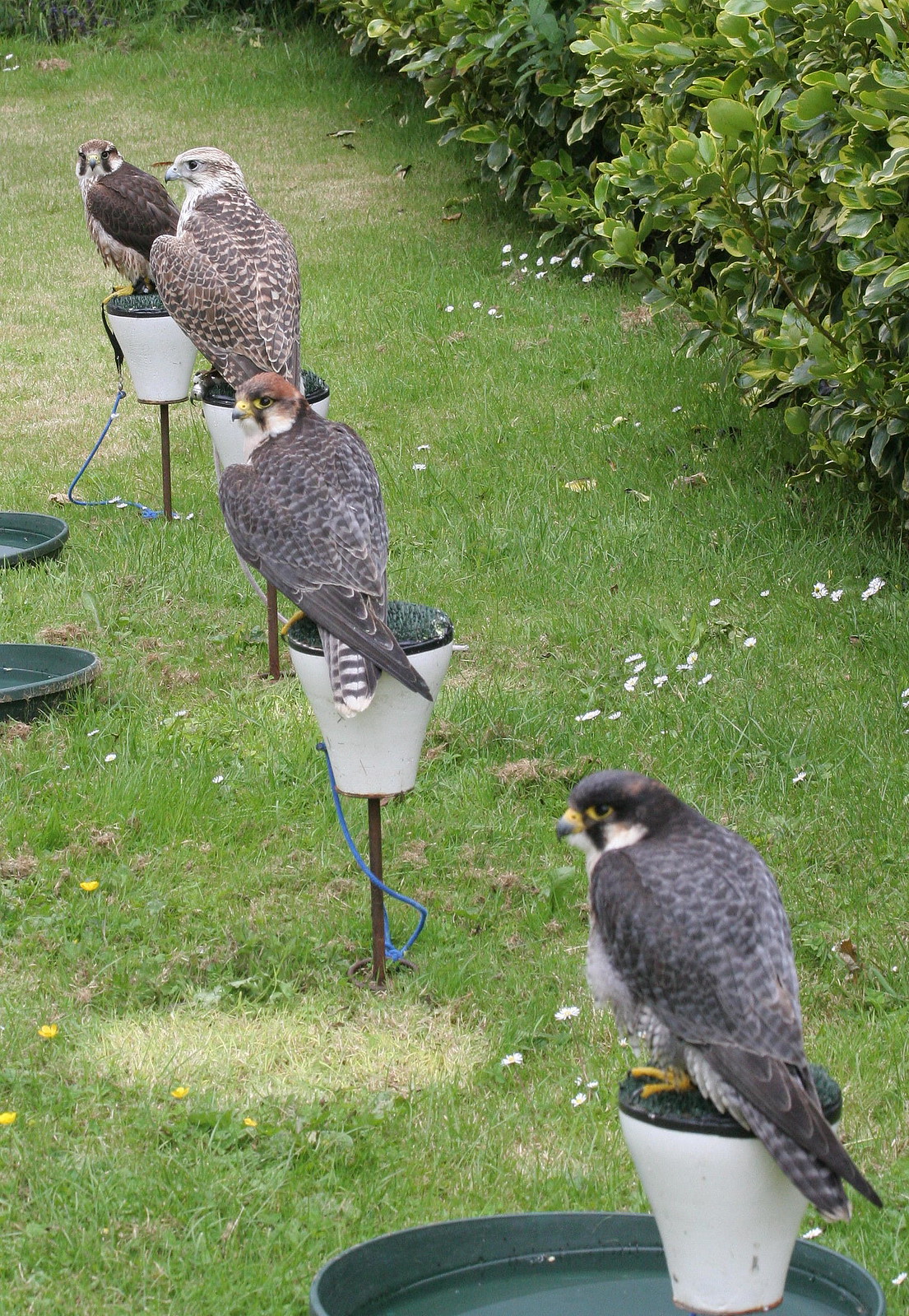The outdoor daytime photograph captures four peregrine falcons and hawks, each perched on white cylindrical stands with green centers, arranged diagonally from the foreground right to the background left. Each bird, viewed in three-quarter profile, has a blue leash attached to one leg, securing them to their respective stands. The birds, distinguished by their short beaks and brown and gray feathers, all face to the left, presenting a coordinated and uniform posture. The ground is covered in lush green grass, and there's a row of green shrubs in the upper right background, suggesting the scene is set in a backyard. One of the birds in the background stands out slightly larger with a lighter head, hinting at individual variations within the species group.